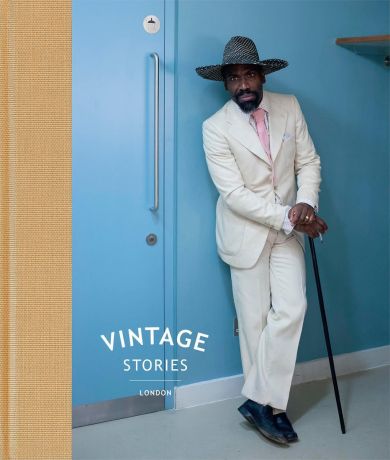The image features an African-American man wearing a sophisticated white suit, complete with a white suit jacket and white pants. He pairs the suit with a light pink tie and a white polo shirt underneath. A stylish dark hat, either black or black and white striped, adorns his head, and he has a black beard. Leaning against a blue wall with a blue door to his right, the man strikes a contemplative pose with one leg crossed over the other, holding a dark-colored cane that he doesn't appear to be leaning on. He completes his ensemble with black shoes.

The blue door beside him has white text at the bottom, which reads "vintage stories" in bold. Below that, and separated by a white line, the word "LONDON" appears in smaller capital letters. The left side of the image features a beige or straw-colored strip, resembling the spine or cover edge of a book, adding to the vintage aesthetic of the scene. The man's stern expression, combined with the vintage-themed branding and stylish attire, suggests a sense of nostalgia and elegance.